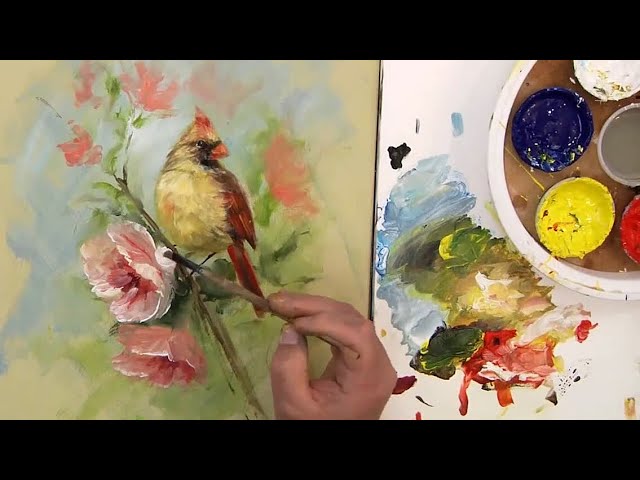In this detailed photograph, we see a close-up of a person's hand holding a brown paintbrush, applying white paint to what appears to be a portion of a flower. The majority of the painting is already completed, featuring a vividly depicted red and yellow bird perched on a branch adorned with pink flowers and green leaves, all set against a yellow background. The bird has a striking red head, a yellow chest, and a bronze-reddish beak. To the right, various open paint cans in white, blue, yellow, and red are visible, positioned on a palette that the artist is using to mix colors. There's also a mixing canvas nearby, displaying splotches of combined colors. The photograph captures both the artist’s meticulous process and the vibrant, almost-complete artwork, framed by black bands at the top and bottom edges of the image.